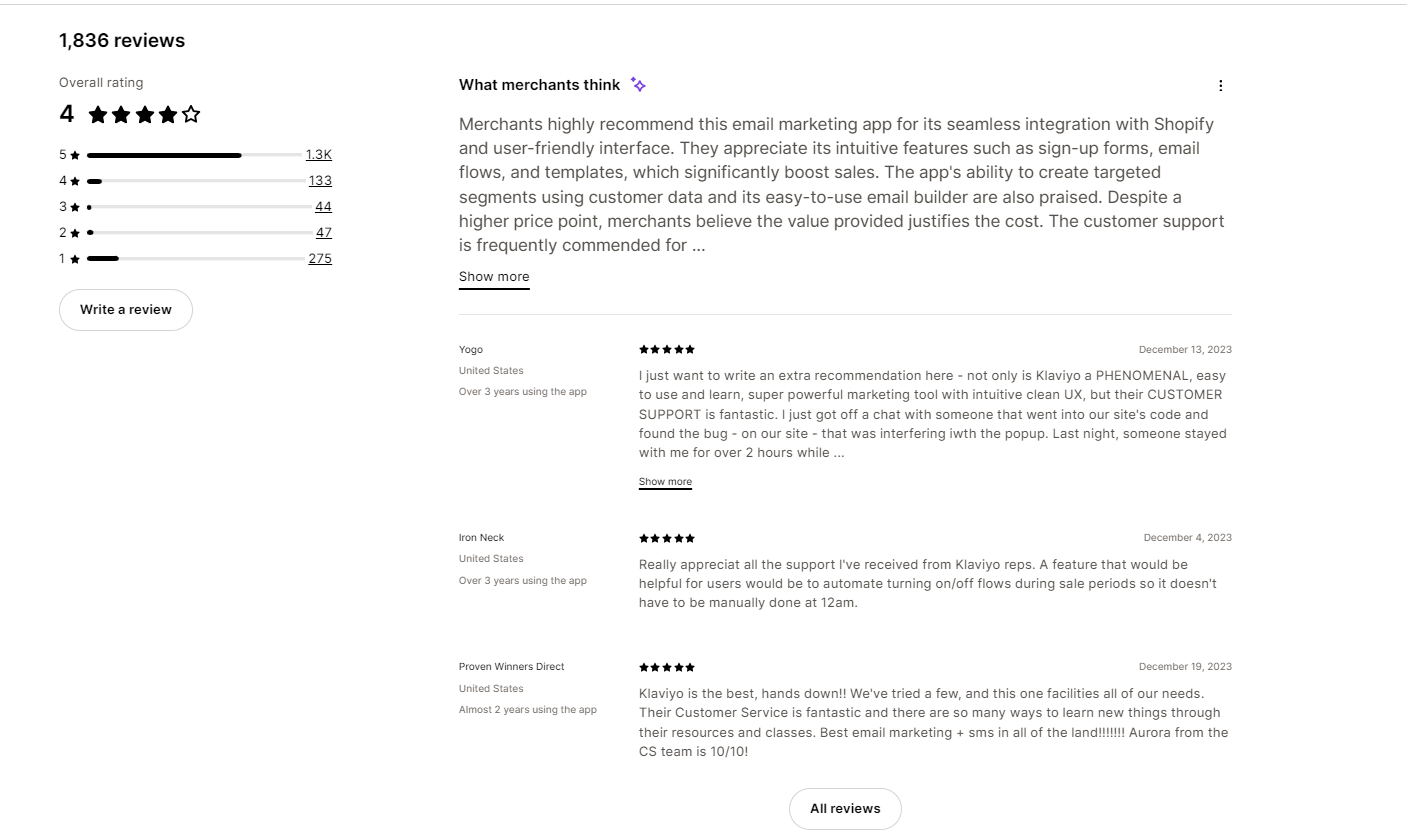In the image, we see a detailed review page for a product or service, showcasing a cumulative rating of four stars based on 1,836 reviews. The reviews are broken down by star ratings as follows: there are 1,300 five-star reviews, 133 four-star reviews, 44 three-star reviews, 47 two-star reviews, and 275 one-star reviews. One highlighted review is by a user named Ionic, who expresses gratitude for the support received from Clavio representatives. Additionally, Ionic suggests a feature improvement for users: an automation option to turn floors on or off during sale periods, eliminating the need for manual adjustments.